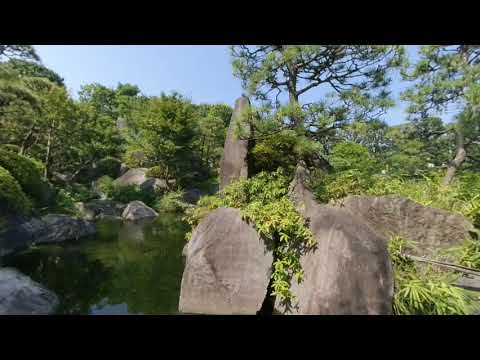This nature photograph captures a tranquil outdoor scene, likely set near the edge of a still, dark green body of water positioned in the bottom left corner. The water is reflective, contributing to the serene ambience. Dominating the foreground are two large, rugged boulders with green foliage clinging to their surfaces, intertwining with ivy and other plant life. These boulders are primarily situated on the right side of the image, creating a stark contrast with the calm water on the left. A rocky hillside ascends from the water's edge, dotted with more boulders and lush vegetation.

In the background, a dense forest encircles the scene, composed of tall trees and bushes in various shades of green, from light to medium tones. The trees are abundant, lending the photograph an untamed wilderness feel. The sky above is a hazy blue, transitioning to a light blue with whitish corners, possibly indicating the presence of sunlight. The overall palette features earthy browns, grays, greens, and hints of blue, reinforcing the image’s natural and untouched atmosphere. This vividly detailed scene evokes the essence of a secluded woodland area, perhaps near a lake, in the middle of the day.